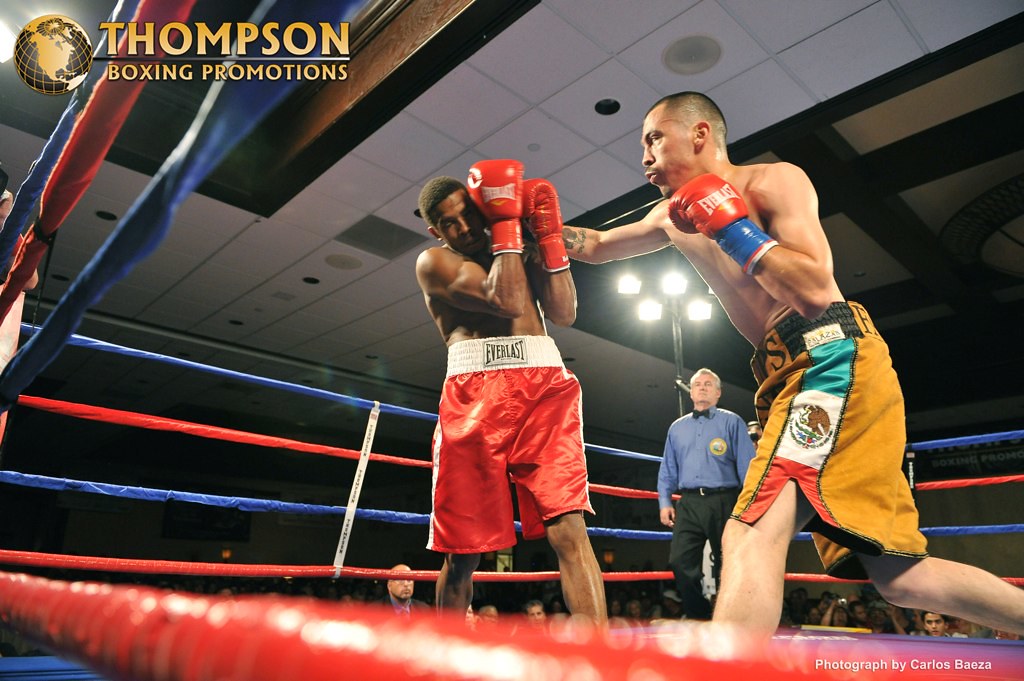In this professionally shot photograph of a live boxing match, we see an intense moment between two boxers at the center of the image. The African American boxer on the left, dressed in red shorts with an Everlast logo, is defending himself with his gloves raised. His opponent, a Hispanic boxer on the right, is mid-punch, wearing gold trunks adorned with the Mexican flag and an Everlast logo on his red gloves. The Hispanic boxer has short black hair and tan skin, and his stance suggests he has the upper hand. In the background, a referee, identifiable by his blue shirt, black bowtie, and short gray hair, watches closely. The scene is framed from a low angle, capturing the ring's red and blue ropes and part of the ceiling with its white tiles and lighting setup. The arena is packed with spectators, though most are dimly lit, with a few in the front row more visible. Above the referee, several lights illuminate the fighters, underscoring the professional nature of the event. The top left corner features the Thompson Boxing Promotions logo and a small credit to photographer Carlos Baeza is visible in the bottom right.